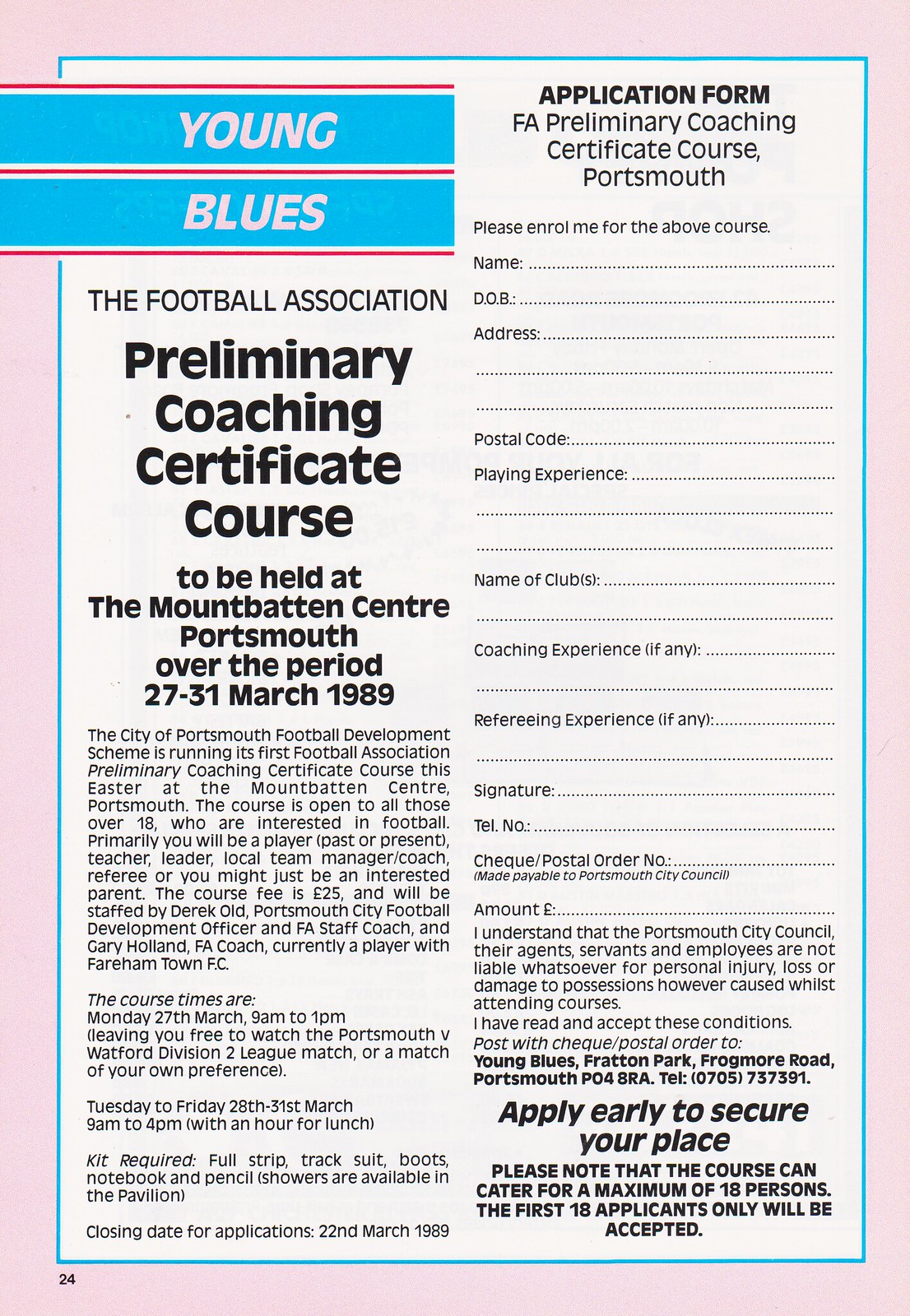The image is an application form for the "Young Blues" Preliminary Coaching Certificate Course, organized by the Football Association, to be held at the Mountbatten Center in Portsmouth from March 27th to March 31st, 1989. The form features a prominent header in white letters against a blue background stating the course details. It is bordered in light pink and includes two main columns. On the left column, the form outlines the course title, venue, and dates. Detailed underneath is a set of instructions and application fields for personal information such as name, date of birth, address, postal code, playing experience, club affiliations, coaching and refereeing experience, phone number, signature, and payment details in Euros. Applicants are prompted to apply early as the course has a maximum capacity of 18 participants, with only the first 18 applications being accepted. Additionally, the form emphasizes understanding and acceptance of the course terms, including liability for injuries. The bottom of the form on the left side is marked with a page number '24'.